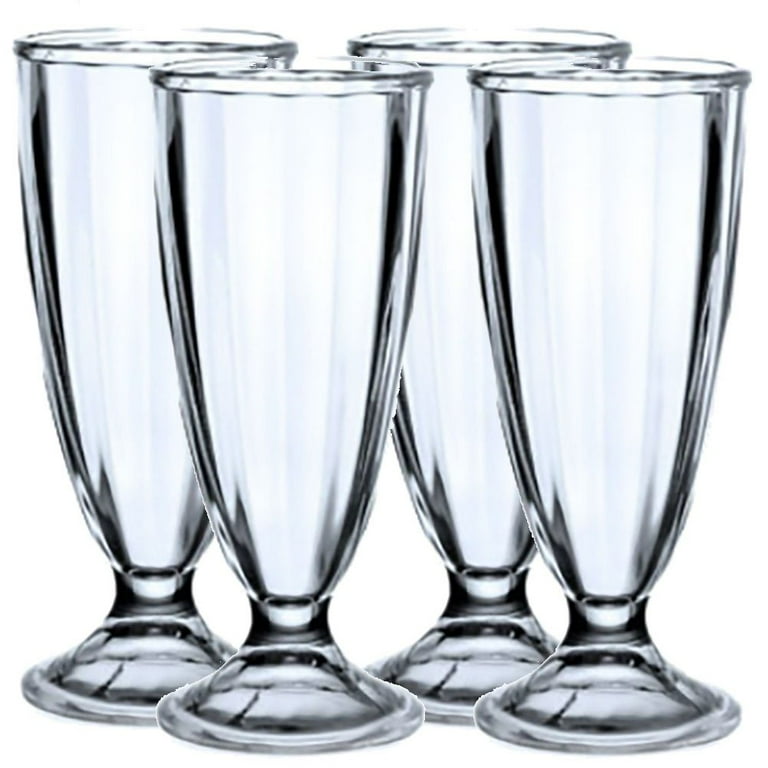This photograph showcases four tall, clear glass dessert glasses arranged against a completely white backdrop. The glasses, which are designed with a circular disc-shaped base, transition swiftly into a wide-mouthed, upward arching U-shape. Though they possess a slight hint of a grayish tint as light refracts through them, they maintain a primarily transparent appearance. Mimicking the base type of a wine glass but without a distinct stem, these vessels are ideal for serving ice cream sundaes or milkshakes. The image is taken at a close-up angle, emphasizing the details and making it suitable for commercial use, like on a website selling these glasses. Arranged in two rows with an alternating pattern, the two glasses in the back are clearly visible through the spaces between the front two, showcasing the elegant, vertical lines that subtly decorate their design. All four glasses are empty and pristinely clean, emphasizing their readiness for use.